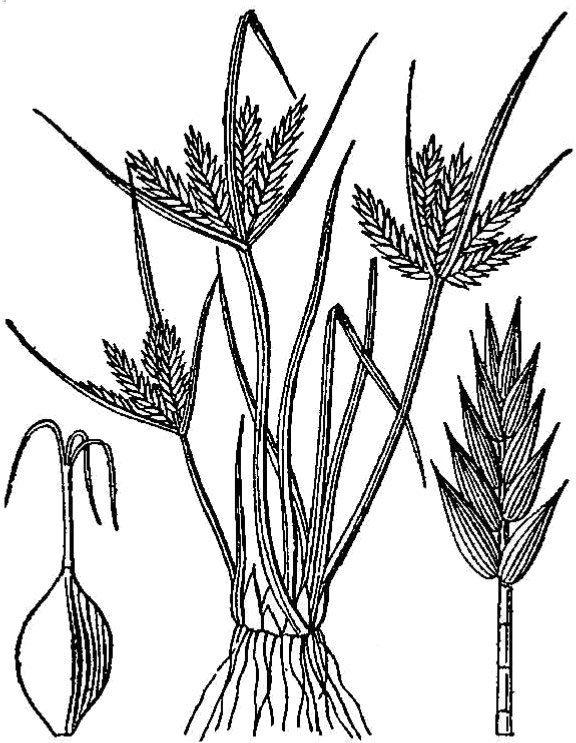This pen and ink drawing on a white background features detailed botanical illustrations of three distinct plants. To the left, there's a plant with an elongated, oval-shaped tuber at the bottom, from which a stem extends upward, supporting three slim leaves that droop downwards. The central illustration depicts a plant resembling wheat, characterized by intricate roots drawn with squiggly black lines beneath it. This plant has basal leaves and long stems that culminate in seed heads akin to wheat's grain clusters, with pointy leaves along the stems, one of which is bent downward. On the right side is a plant whose upward-pointing stems and leaves give it a tree-like appearance, with clustered elements that might resemble ears of corn or seed heads.